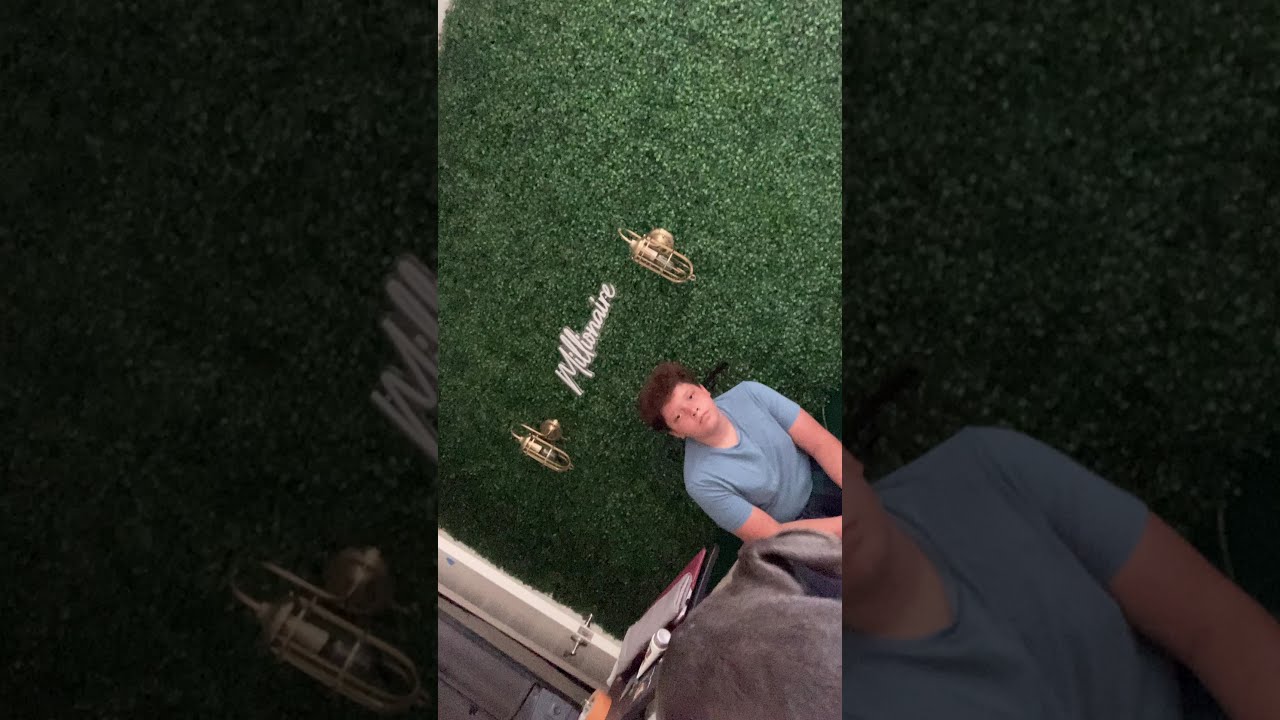The photograph is divided into three vertical sections, with the first and third sections featuring darkened close-up images of the middle section. The middle section shows a young boy with fair skin and brown curly hair, wearing a light blue t-shirt, sitting on what appears to be green grass, though it seems to be artificial. The boy is positioned slightly tilted, and he gazes directly at the camera with a neutral expression. Behind him, there is a backdrop that looks like a wall made of greenery, possibly artificial plants. Flanking the boy's head are two golden sconces, resembling wall decor or light cages. Between the sconces, the word "Millionaire" is illuminated in white neon script. The overall image gives an impression of being indoors, and there’s a subtle reflection of the boy in the lower part of the picture, suggesting a mirror might be involved.